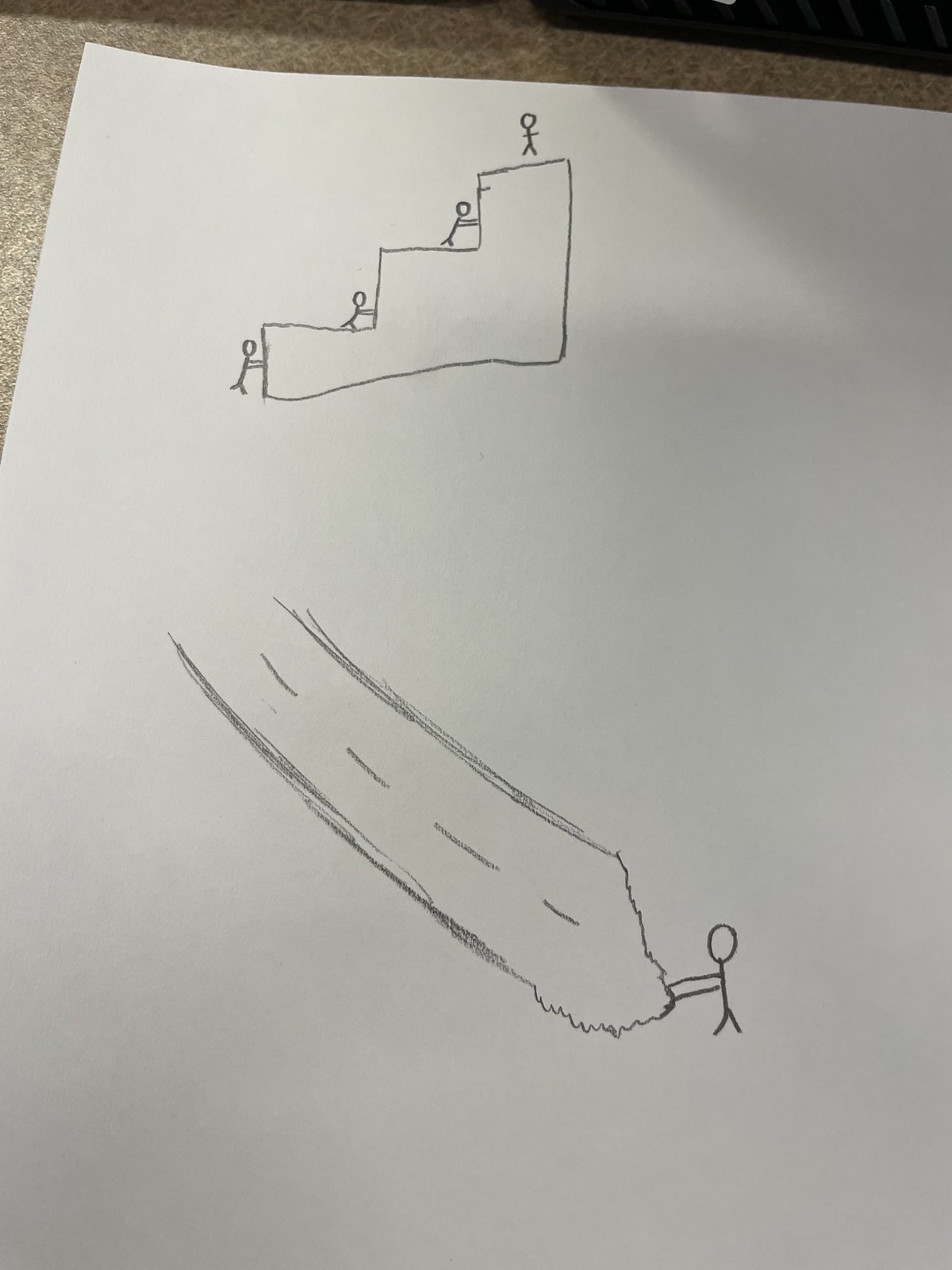This detailed and expressive child's pencil drawing is sketched on a sheet of white paper, which rests atop a beige table. Dominating the top portion of the artwork are three towering steps that dwarf the small stick figures attempting an ascent. Each step is significantly taller than the figures themselves, creating a challenging and dramatic climb. Positioned strategically, a stick figure stands at the base, while another figure halfway ascends the first step. Another figure reaches the second step, pushing against its daunting height, and finally, a triumphant figure with outstretched arms stands atop the third step in a gesture of victorious accomplishment.

Below this striking scene, the drawing transitions to depict a piece of road being lifted and dragged by yet another stick figure. The distinctive stripes that typically mark the center of a road are clearly visible, adding a touch of realism to the whimsical scene. The stick figure, bent in effort, appears to have uprooted a section of the road and is in the process of pulling it along.

Overall, this imaginative drawing combines elements of struggle, determination, and victory through the simple yet powerful depiction of stick figures in various states of action and achievement.